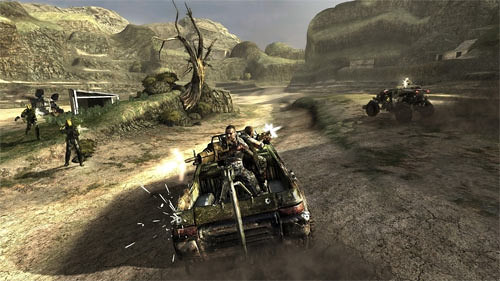This scene is a screenshot from the video game "Haze," released around 2007-2008 by Ubisoft. The image, rectangular and small, vividly captures a war zone scenario set in a sandy area surrounded by towering rocky mountains. In the foreground, a military truck with a mounted machine gun is prominently displayed. A soldier manning the gun in the back of the truck is firing off to the left, sending visible bullet streaks hitting just above the taillight. Inside the truck, another person is in the front seat, also equipped with a mounted machine gun, aiming at an ATV-like vehicle to the right. Additional soldiers are scattered around to the left, enhancing the chaotic battlefield atmosphere. In the far left background, an overturned vehicle adds to the scene's intensity, while a small hut perched on a rocky ledge can be seen to the right. The rugged, rocky terrain and sparse grassy patches complete this detailed depiction of the in-game war zone.